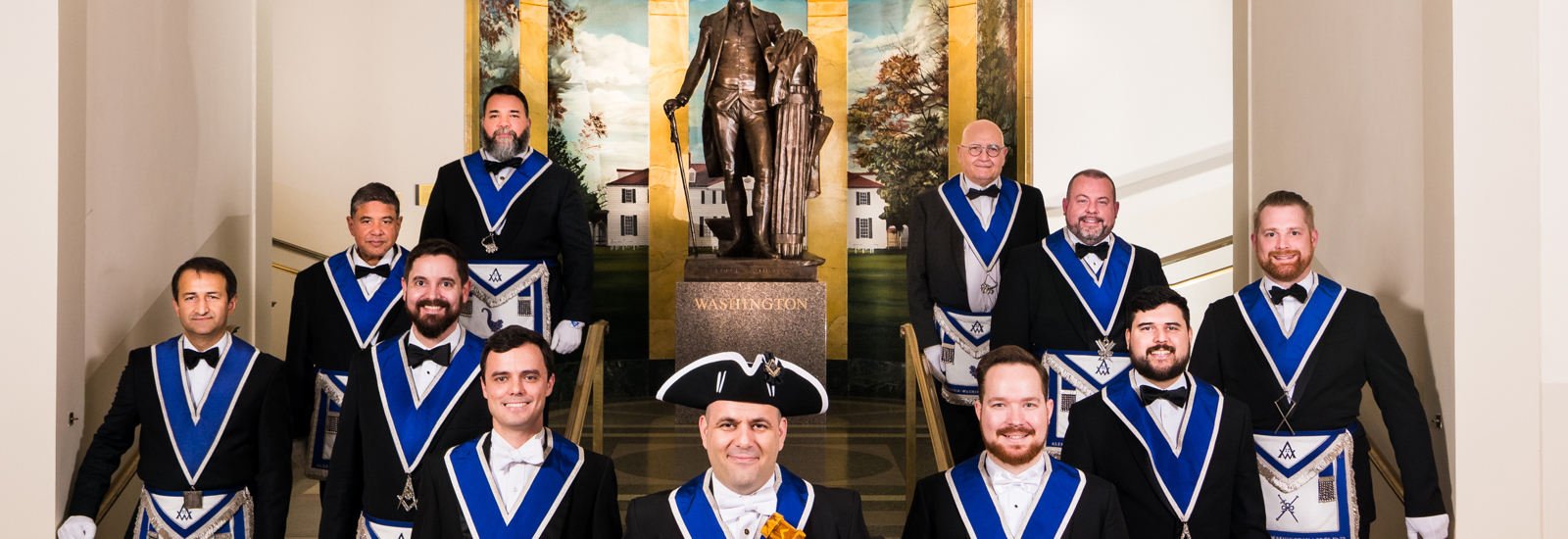The image portrays a formal portrait of a group of nine men, presumably Freemasons, dressed in black suits with white collared shirts and bow ties—most in black bow ties, but three in the front wearing white ones. Each man dons a blue v-neck medallion featuring the silver Mason's logo, and some wear crowns or medallions. One central figure at the bottom stands out, wearing a distinctive old-school army hat, resembling an upside-down taco shell or a pirate hat with white trim. They are posed indoors, in what appears to be a gray-walled convention or ceremonial setting, around a central staircase. Dominating the background is a tall, bronze statue labeled "Washington" on its stone base in yellow text, where the bronze figure leans on a pillar. The photo is landscape-oriented, focusing on the group from the shoulders up, and captures the men forming a semi-circle around the statue, signifying their organized and formal gathering.